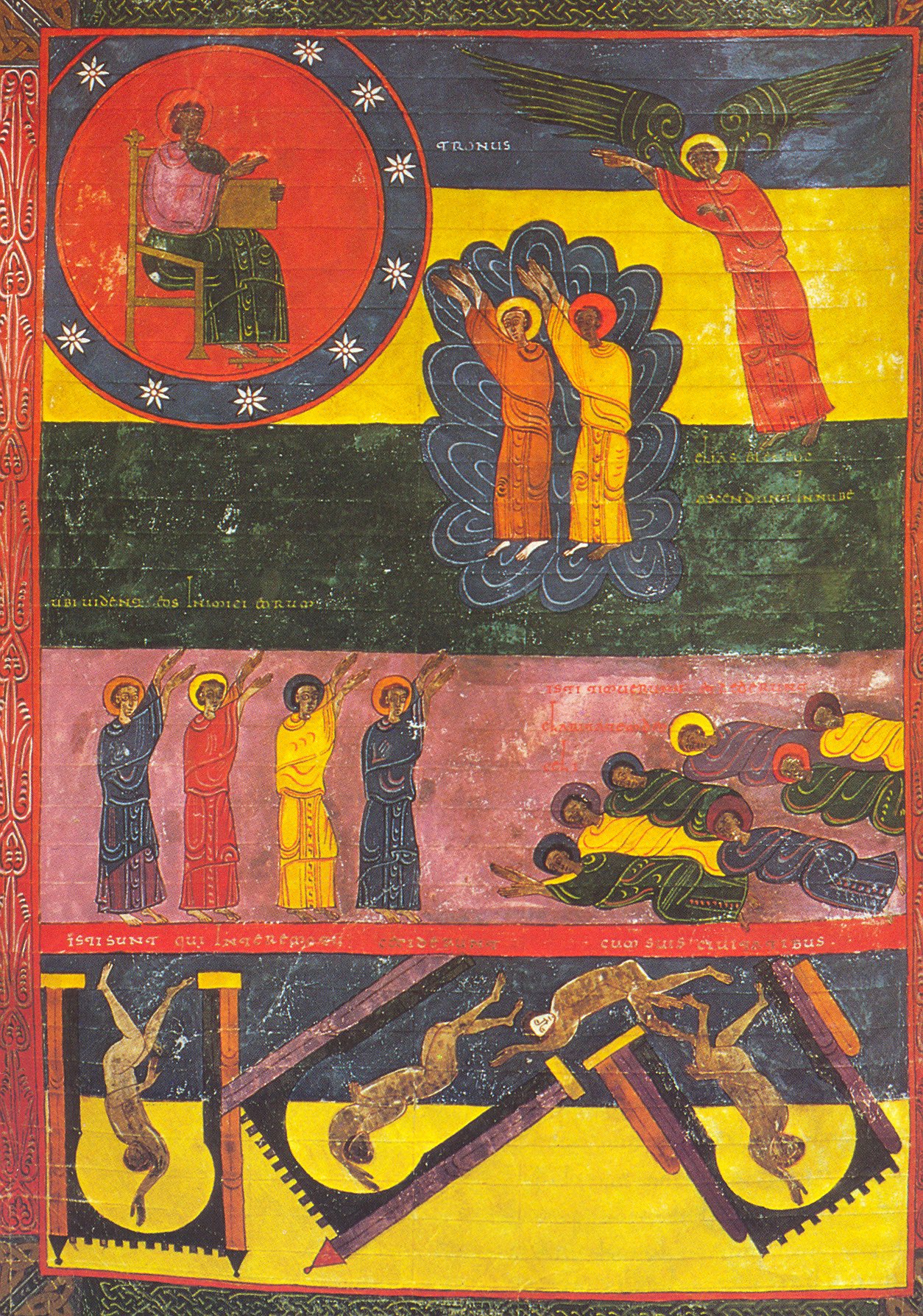The artwork is a vivid and textured mural, possibly painted on a brick wall or a stone surface, showcasing a tapestry of colors that include reds, blues, yellows, and blacks, with hints of oranges and muted greens. Dominated by religious themes, it features dark-skinned figures in foot-length robes of red, yellow, orange, pink, black, and blue. The painting is divided into five distinct levels, each narrating a different part of a collective spiritual journey.

At the top left corner, a central figure, possibly a woman, seated in a red circle, holds what appears to be a musical instrument or a script, suggesting significance or authority. Beside her, several figures, appearing to worship her, raise their hands—one of them adorned with angelic wings, elevating slightly above the others.

Beneath this heavenly scene, the subsequent levels show more figures in reverence, some raising their hands in worship, while others lay lifeless or in prayer, hinting at a passage or transition. The lower portion appears chaotic; some figures lie naked as if expelled from grace, resembling an interpretation of purgatory or hell. Strangely shaped entities at the very bottom, possibly depicting dead bodies or fantastical creatures, are confined within what looks like rotating gates.

A red and black border with a silver pattern adds to the structured yet chaotic composition, and the painting is segmented with stripes of red-bordered sections at both the top and the bottom, containing blue, yellow, black, and pink tones above, and black and yellow stripes below. The entire artwork appears to be delicately folded and unfolded, suggesting it might have been a portable piece displayed for worship or judgment scenes.